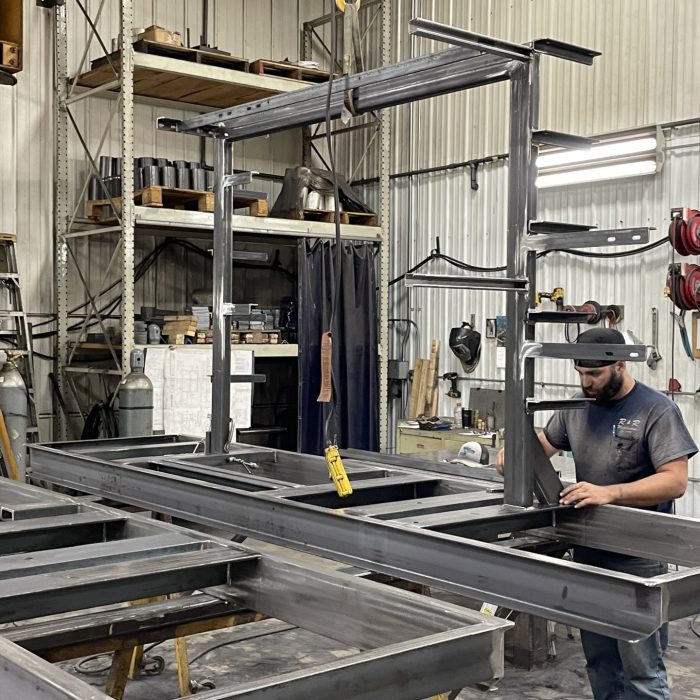In this photograph, a man with light to medium skin and a black beard is working in a meticulously organized metal workshop with white aluminum walls, which gives the appearance of a Quonset hut. He is wearing a gray t-shirt and a gray cloth cap that resembles a surgeon's cap, and he has a blue pen with "R&R" above his shirt pocket. The man appears to be staging a metal frame for welding, as indicated by the various discolored welding points on the metal pieces.

Front and center in the image are two rectangular, flat steel tables with openings separated by bands of steel. One table in the middle features a prominent steel arch frame overhead from which various cables hang, including a yellow and a tan item. The man stands to the far right, holding a black object at the edge of this table.

The workshop is well-equipped, with metal storage racks on the left side full of silver, gray, and brown metal components stacked on wooden platforms. A black curtain is pulled to the right, exposing the middle shelf of the storage rack. Also on the left are two oxygen tanks and an aluminum ladder leaning against the wall.

The walls are adorned with various tools and brackets, creating an industrious atmosphere. A red pulley system and a fluorescent light fixture with two bulbs are visible behind the man. Tools such as wrenches, saws, and a drill, as well as a welder's mask, are hung on the walls, indicating a space designed for intricate metalwork and welding tasks.